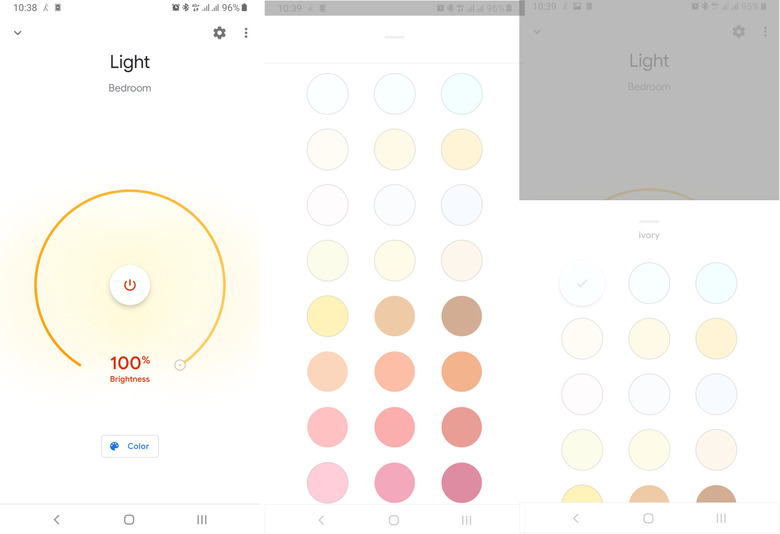This image displays a screenshot taken from an Android device, showcasing multiple layers of details. There are three individual screenshots within the main image, each providing a comprehensive view of the phone's interface. 

At the top left corner of all screenshots, the current time is clearly visible. Adjacent to this, a series of icons indicate various notifications and status alerts: an alarm notification icon, the Bluetooth symbol, and network signal indicators for SIM 1 and SIM 2. Additionally, the top right corner of the status bar features a patch level indicator.

The screenshots are vibrant with a spectrum of colors ranging from bright white to deep brown and delicate shades of pink, creating a visually appealing contrast. 

In the center of the first screenshot, prominently displayed is a switch button. Just below this central button, the screen showcases a brightness level indicator set at 100%, ensuring maximum screen visibility.

Overall, this detailed depiction beautifully captures the intricate elements and functionalities of the Android device’s interface.